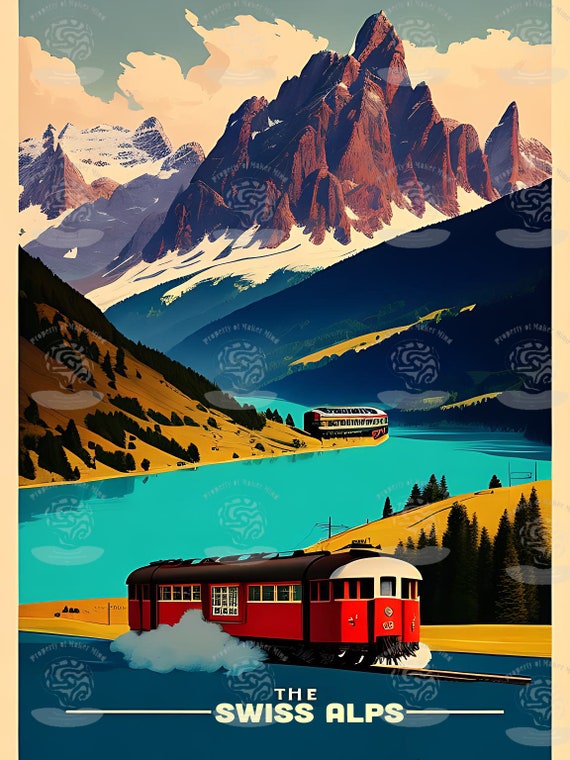The image, reminiscent of vector art and graphic design, serves as an advertisement for the Swiss Alps. The word "The Swiss Alps" is prominently displayed in white text at the bottom, flanked by small white bars on either side. Dominating the lower section of the image is a lone red train car with a black roof and a white front roof, running on rails. Puffs of smoke or snow trail from the sides of the car. Behind the train, a yellow hill dotted with green pine trees slopes down to a vibrant blue body of water. As you ascend the image, the scenery transitions to a rugged mountain range with jagged brown cliffs and snow-covered peaks. Above lies a misty, teal-colored sky filled with thick, yellowish-tan clouds. A watermark, featuring a brain-like logo and the text "property of maker," is repetitively stamped across the image, emphasizing its digital creation.